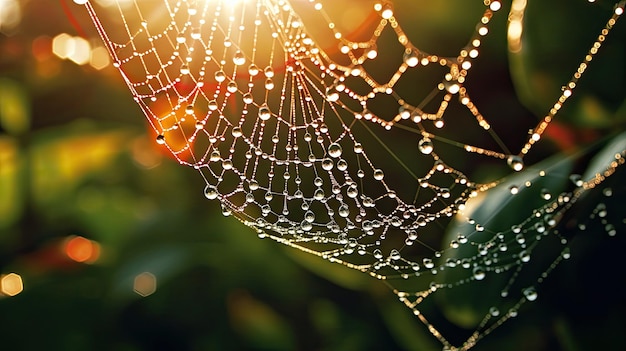The focal point of this outdoor image is a large, intricate spider web adorned with numerous water droplets that glisten where the web's strands intersect, particularly in the square patterns. The web occupies the forefront of the image, appearing almost like a lacework of light and moisture. The bottom portion of the web forms a distinct triangular shape, adding an interesting geometric element to the scene. The background is heavily blurred, creating a bokeh effect with a mix of green foliage and varying hues of yellow and orange, suggestive of plant life. Sunlight filters through, causing parts of the background to glow with white, red, blue, and orange highlights. In the foreground, a few leaves, more defined in focus, contribute additional green and yellow tones. The interplay of sunlight through the droplets on the web further enhances the overall ethereal quality of the image.